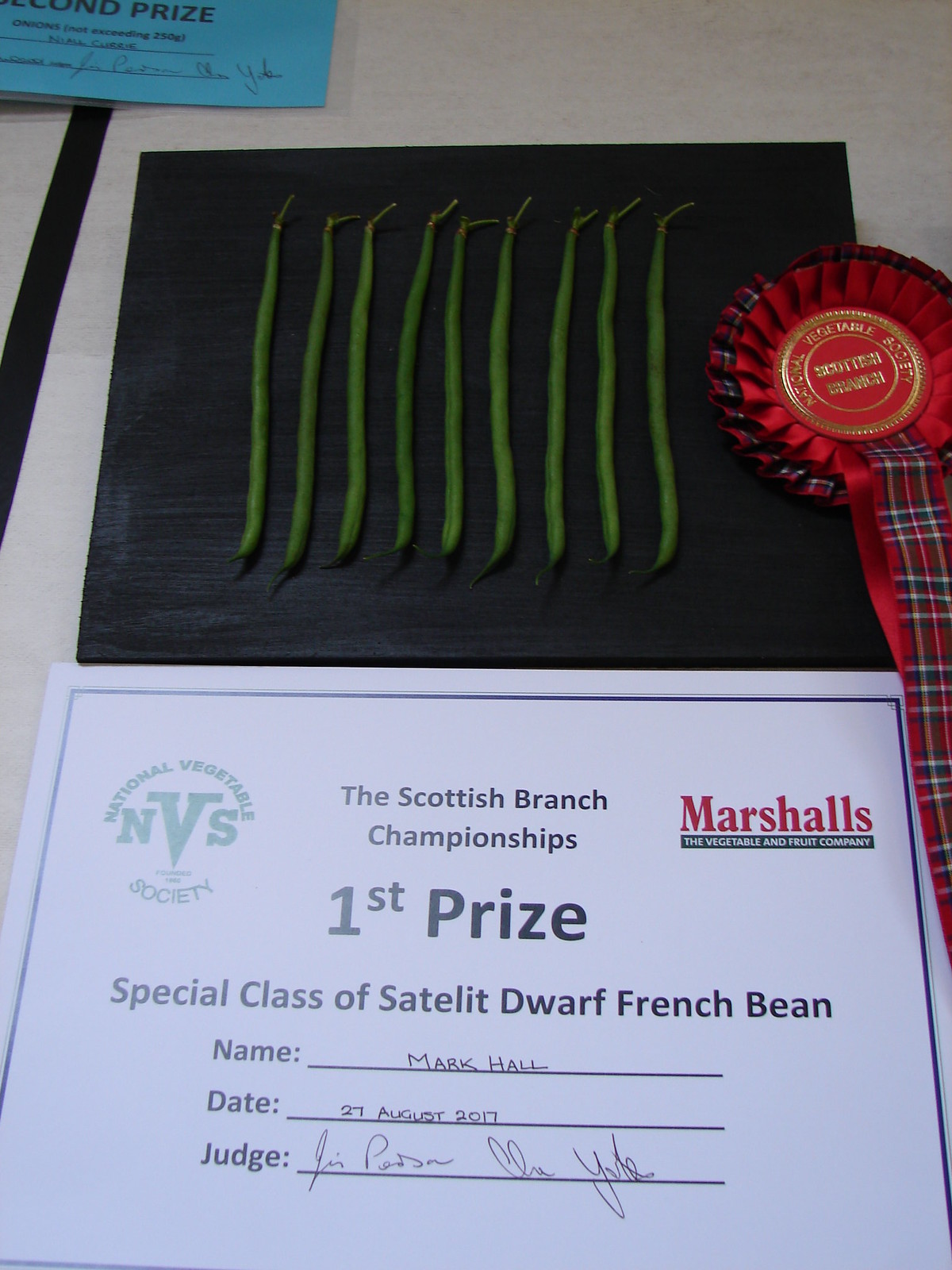This detailed photograph depicts an award display from the Scottish Branch Championships, held on August 27, 2017. The centerpiece of the image is a white certificate with black lettering, awarded to "Mark Hall" for securing the First Prize in the Special Class of Satellite Dwarf French Bean. The certificate prominently features the MBS Society logo on the left and the Marshals logo on the right, indicating sponsorship. This certificate rests on a beige wooden table.

Just above the certificate, a blackboard displays nine neatly aligned green beans, placed vertically to showcase their full length from stem to tip. To the right of the beans, a bright red ribbon is visible, highlighting the award's significance. Lying on a white background, the certificate adds contrast to the vibrant colors surrounding it, with shades of tan, off-white, black, light blue, red, green, and white present in the scene.

In the top left corner of the photograph, there is a partial view of another certificate, blue in color, suggesting it might be a second prize award, though less prominently featured. The image captures the essence of an indoor award ceremony, celebrating agricultural excellence.